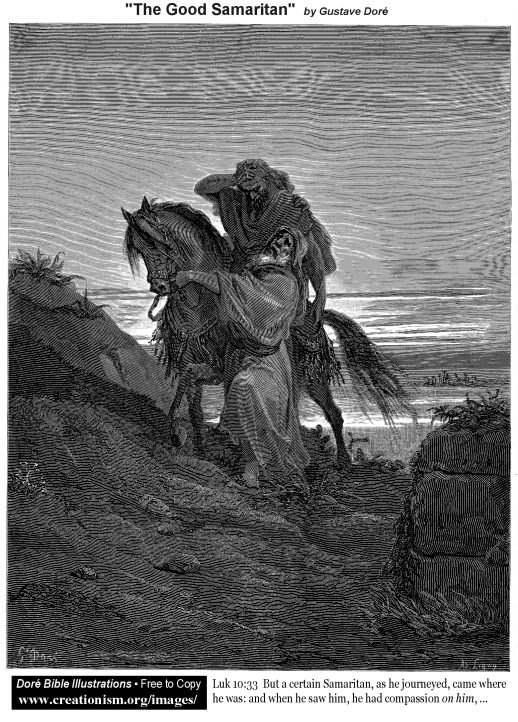This black-and-white image, showcasing Gustave Doré's engraving titled "The Good Samaritan," features intricate detailing created through finely etched lines. Central to the piece is a poignant scene from the biblical story: an older man with a white beard, dressed in a draping robe, kneels beside a horse, holding it in an embrace. This older man appears compassionate and is aiding another man who is mounted on the horse. The man on the horse, also wearing a robe but in darker shades, holds his head in what seems to be pain or distress and has long hair cascading over his shoulders. The landscape slopes uphill with rocky, grainy soil, giving the impression of an arduous journey. In the background, a short stone wall is visible to the right, leading to a flat stretch of ground that melds into the horizon. The engraving includes a textual header reading “The Good Samaritan” by Gustave Doré, and a footer stating, “Doré Bible illustrations, free to copy” with the URL and the biblical passage from Luke 10:33: "But a certain Samaritan, as he journeyed, came where he was, and when he saw him, had compassion on him."